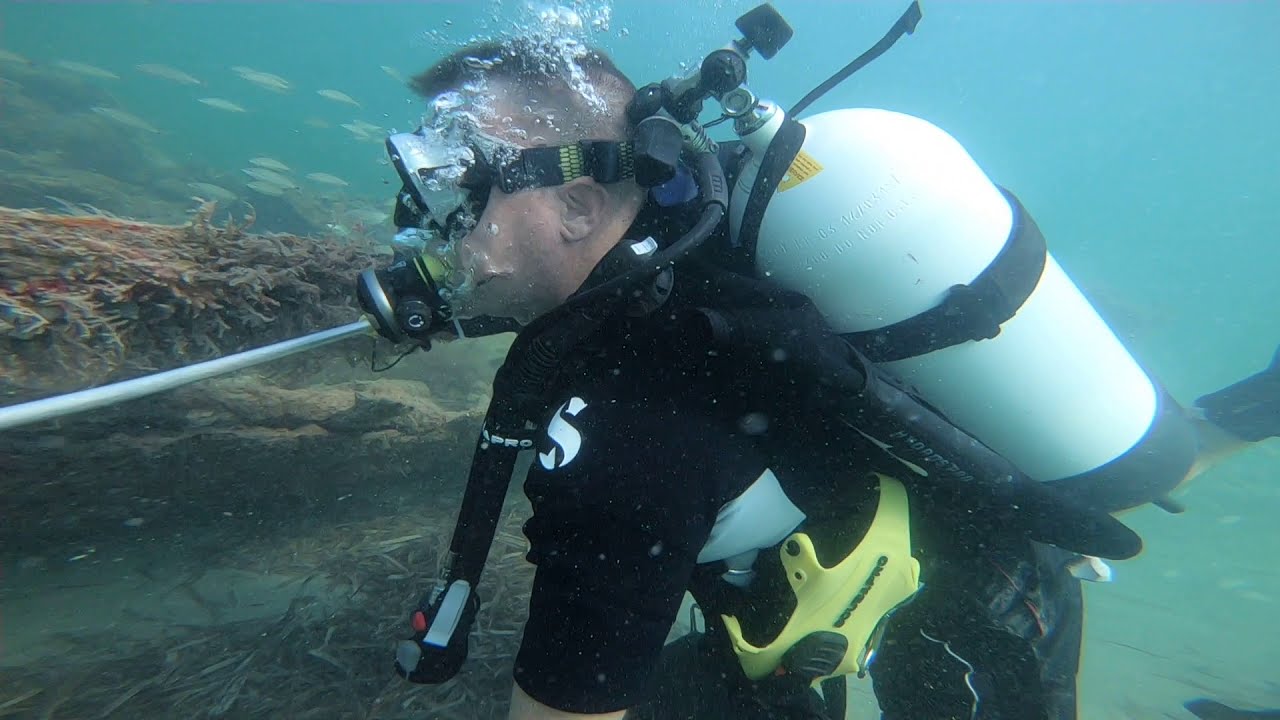The detailed underwater photograph features a man wearing scuba gear, including a black wetsuit with white trim and goggles that cover his eyes. He is facing slightly to the left and has a white oxygen tank strapped to his back, along with a yellow apparatus on his waist. His face is surrounded by numerous bubbles, and he sports a spiky military-style haircut. The diver occupies the center of the image, almost stretching from top to bottom.

In the background, to his left, there is a rock formation adorned with brown seaweed. A school of small, dark yellowish fish can be seen swimming around the reef and behind the diver. The water appears somewhat murky but is well-lit from above, allowing clear visibility of the various elements in the scene. Lastly, a variety of colors such as red, brown, tan, yellow, white, black, pink, and gray are subtly present throughout the image, adding to the visual complexity of this underwater snapshot.